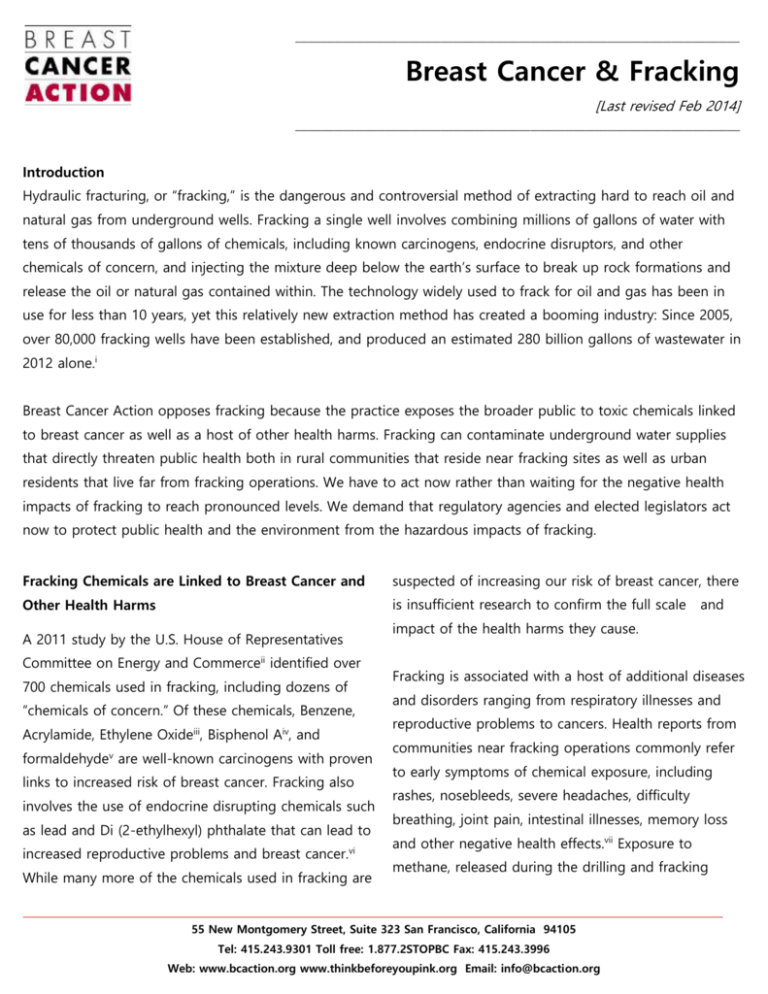The image features an article produced by an organization called Breast Cancer Action. In the top left corner, there is a black horizontal line followed by the word "BREAST" in a thin, rounded sans-serif font with prominent character spacing. Another black-bordered line follows, leading to the word "CANCER" in bold, uppercase black lettering. Below this, a somewhat faded black divider appears. Subsequently, the word "ACTION" is displayed in even bolder, red uppercase letters, which is once again followed by another black divider.

On the right side of the page, there are two long horizontal dividers extending through more than half the page. Beneath these dividers, centered in bold black text, the title "Breast Cancer and Fracking" is presented. Directly underneath this title, in small, italicized black text enclosed in brackets, is the revision date "Last revised FEB 2014."

The body of the article begins with the word "Introduction" in bold, small black lettering towards the left. This is followed by two paragraphs of non-bold, black text discussing the introductory topic and subject matter.

Towards the bottom left of the page, a new header in bold black text reads "Fracking Chemicals are Linked to Breast Cancer and Other Health Harms." This section contains two additional paragraphs: the first paragraph starts on the left and flows into the right column, leading into the second paragraph.

At the very bottom of the page, there is a single orange horizontal line divider.